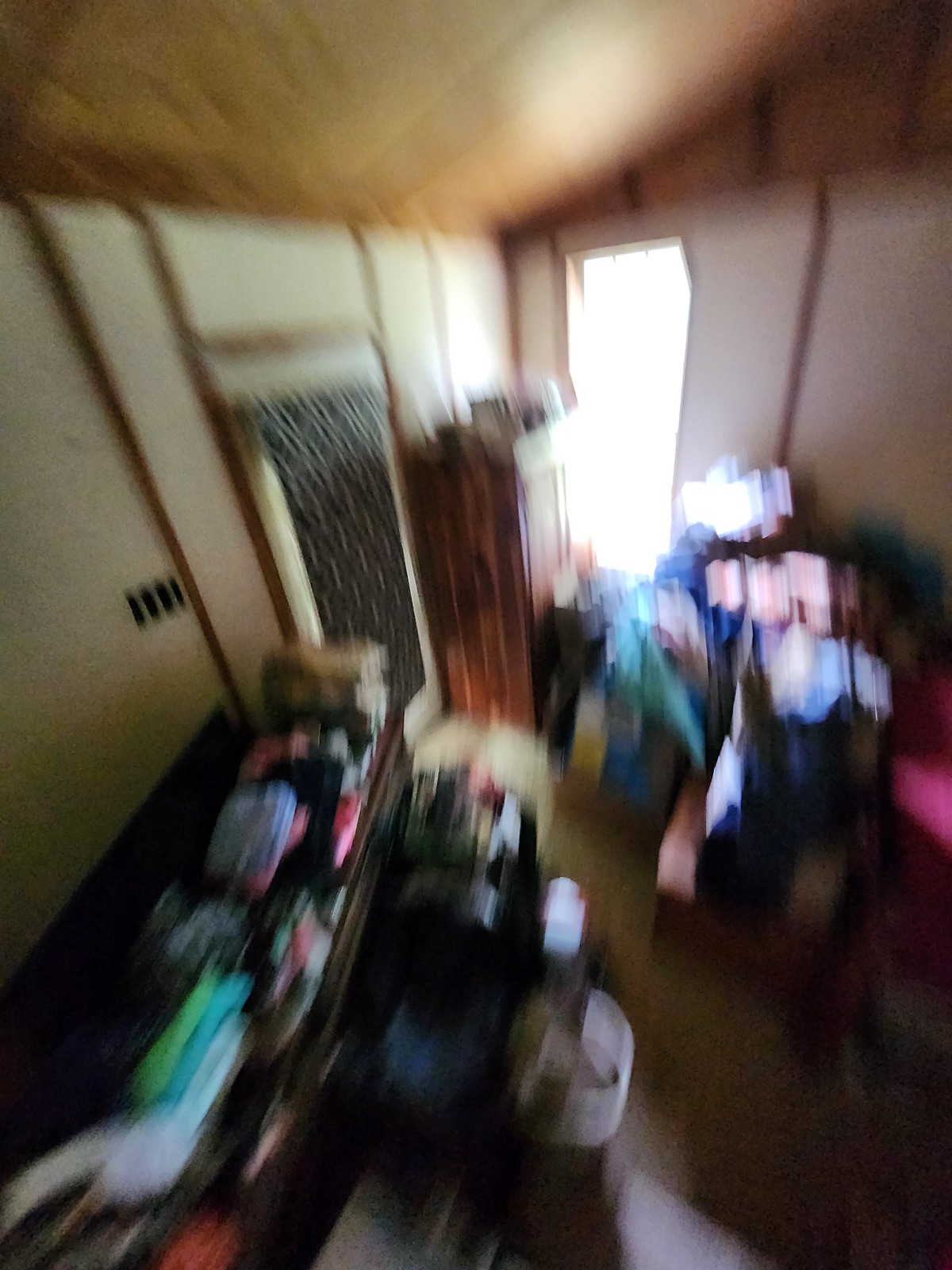The photograph depicts a cluttered room that is possibly a closet or a bedroom. The space is filled with an array of clothing and other items scattered throughout, creating a somewhat chaotic scene. The image is slightly blurred, making it difficult to discern specific details but allowing the viewer to note the general color scheme. On the right side, shades of blue, pink, and white are predominant, while the left side features hues of green, black, pink, and white. The walls are a tan color, accentuated by a brown wood trim that outlines the doors and windows, adding a touch of warmth to the room's aesthetic. The slanted ceiling, composed of brown wood, complements the overall color palette. A bright light streams in from a window on the back wall, illuminating the space. Centrally placed in the room is a medium-toned brown wardrobe, with various indistinct items perched on top.